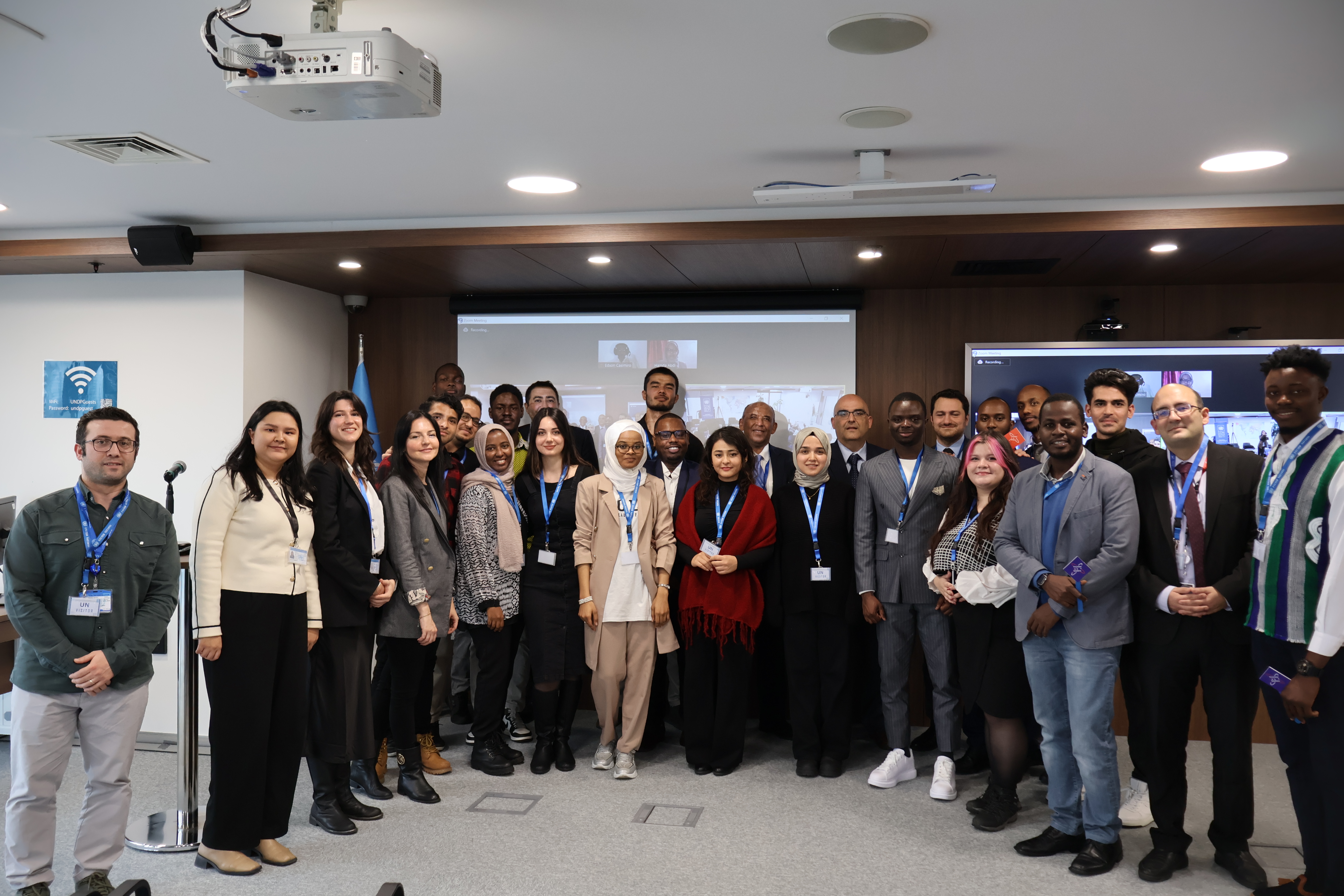This color photograph captures a diverse group of approximately 20-32 professionals standing in a semicircle inside an office setting, likely during a conference or event. The attendees, a mix of men and women of various ages and ethnicities, are all wearing blue lanyards with white badges around their necks. They are positioned in front of two large projector screens, one of which is displaying a Zoom call. Some distinct individuals include a woman with a head covering and another with pink hair, reflecting the group's diversity. 

The room features a white ceiling with recessed lighting and a brown wooden accent wall at the back. A projector is mounted on the ceiling, casting an image onto one of the screens. A microphone stand is visible on the left side of the image, placed between the two leftmost attendees. The floor is carpeted in gray and a blue Wi-Fi symbol is visible on the left wall. Everyone is dressed in business casual attire, presenting a professional yet approachable image. Most attendees are smiling, exuding a positive atmosphere indicative of a celebratory occasion, such as the "Frontier Tech Leaders" first machine learning boot camp graduation.